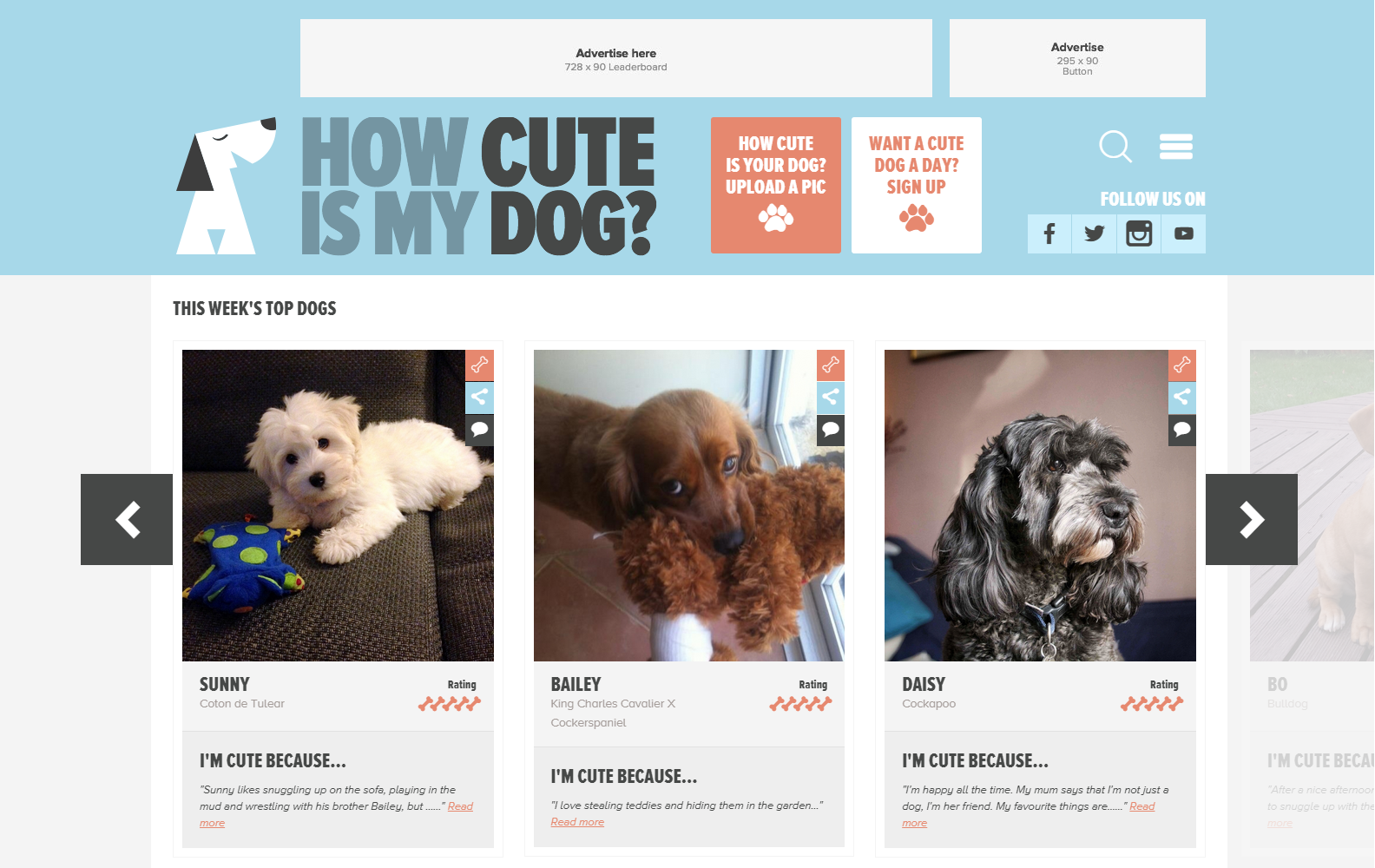**Screenshot Description:**

The screenshot features a vibrant webpage titled "How Cute is My Dog?" The left side of the title showcases an animated white dog facing right, characterized by a triangular black ear and a black nose, with the art style comprising sharp edges. 

To the right of the title, there are two interactive boxes. The first, in red with white text, prompts users with "How Cute is Your Dog? Upload a pic" and includes a white paw print icon. The adjacent box is white with red text, reading "Want a Cute Dog a Day? Sign up," and it also features a red paw print icon. 

Above the main title, the light blue header includes social media buttons for Facebook, Twitter, Instagram, and YouTube. Additionally, there are two banner ads: one rectangular ad stating "Advertise Here," and another smaller rectangle with dimensions marked as 208 by 90.

The body of the webpage displays three adorable puppy pictures. 

1. **Sunny**: A white medium-furred dog sitting on a black couch.
2. **Bailey**: Likely a Cocker Spaniel, this brown-furred puppy holds a curly brown plush toy in its mouth.
3. **Daisy**: A Cockapoo breed featuring long hair and floppy ears with a notable five-star rating (depicted using bones).

Each puppy image is accompanied by a five-bone rating and a brief description about the dog underneath the ratings.